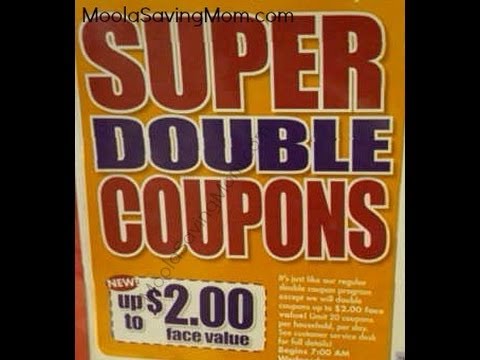The image is a horizontal rectangular picture of a sign set against a pure black background. The sign has an orange background, featuring bold text in three different sections. At the top, the word “SUPER” is displayed in large red letters with a yellow border. Beneath it, “DOUBLE” is written in slightly smaller gray letters, also bordered in yellow. The word “COUPONS” appears in large red letters with a yellow border at the bottom. Within the bottom left corner of the sign, there's a red circle with the word "NEW" and additional text stating "up to $2 face value," with "$2" prominently in large font above the smaller "face value" text. On the right side of the sign, there's a chunk of yellow text, too small to easily read, spanning around 10 lines. At the top left corner of the image, the website "moolahsavingmom.com" is visible. The sign is outlined with black bars framing it on either side.